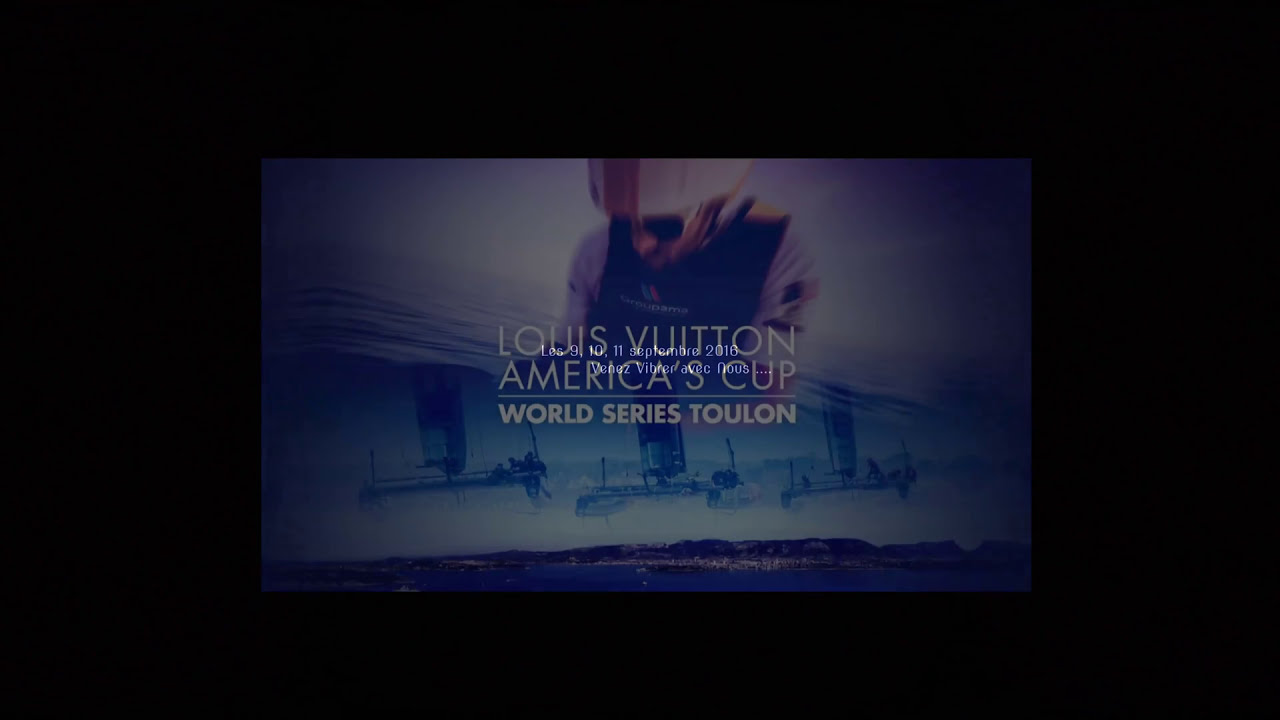The image is a promotional panel for the Louis Vuitton America's Cup World Series Toulon. The background is predominantly black, while the foreground features a screen displaying text that reads "Louis Vuitton America's Cup World Series Toulon" in white letters. At the top center of the screen is a close-up of a man from the chest up. He is wearing a white helmet with a red stripe down the center, black sunglasses, and a black vest over a white shirt. An American flag insignia is visible on his left arm. Below him are scenes of the event. One part depicts fast-moving catamarans with their sails up, floating on blue ocean water, contrasted against a scenic harbor filled with docked boats, trees, and buildings. The sky above the harbor transitions from light to dark blue, suggesting different stages of the day.